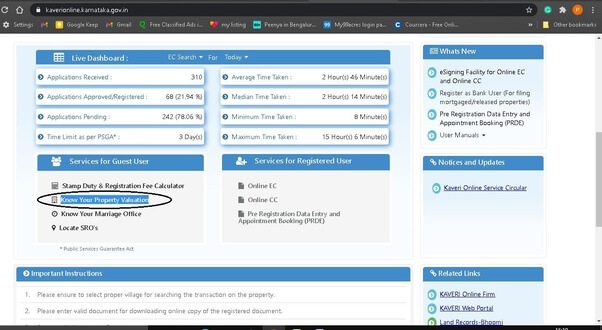An image depicts a bustling web page brimming with functionalities and options. The top section features a search bar labeled “Klarna Market” alongside icons for settings, refresh, home, and a lock symbol, indicating secure browsing. Various colorful icons represent Google Maps, Gmail, and free classified ads, accompanied by tabs and bookmarks for frequently accessed sites. Unfamiliar symbols, including an aqua icon, a clip-like symbol, and an orange icon possibly linked to social platforms like Twitter or Instagram, add to the array. A trio of dots hints at more options or a help menu.

The central part of the webpage showcases a “Live Dashboard” headline, emphasizing “easy search for today” with eight selectable options. Segments such as "Services for Guest User," "Services for Registered User," "What's New," and "Notices and Updates" structure the content, inviting users to explore various services and news updates.

At the bottom, sections for “Important Instructions” and “Related Links” provide additional resources and guidance. The layout suggests a comprehensive and user-friendly interface, ideal for learning and quick navigation, making it a practical home base for frequent exploration.